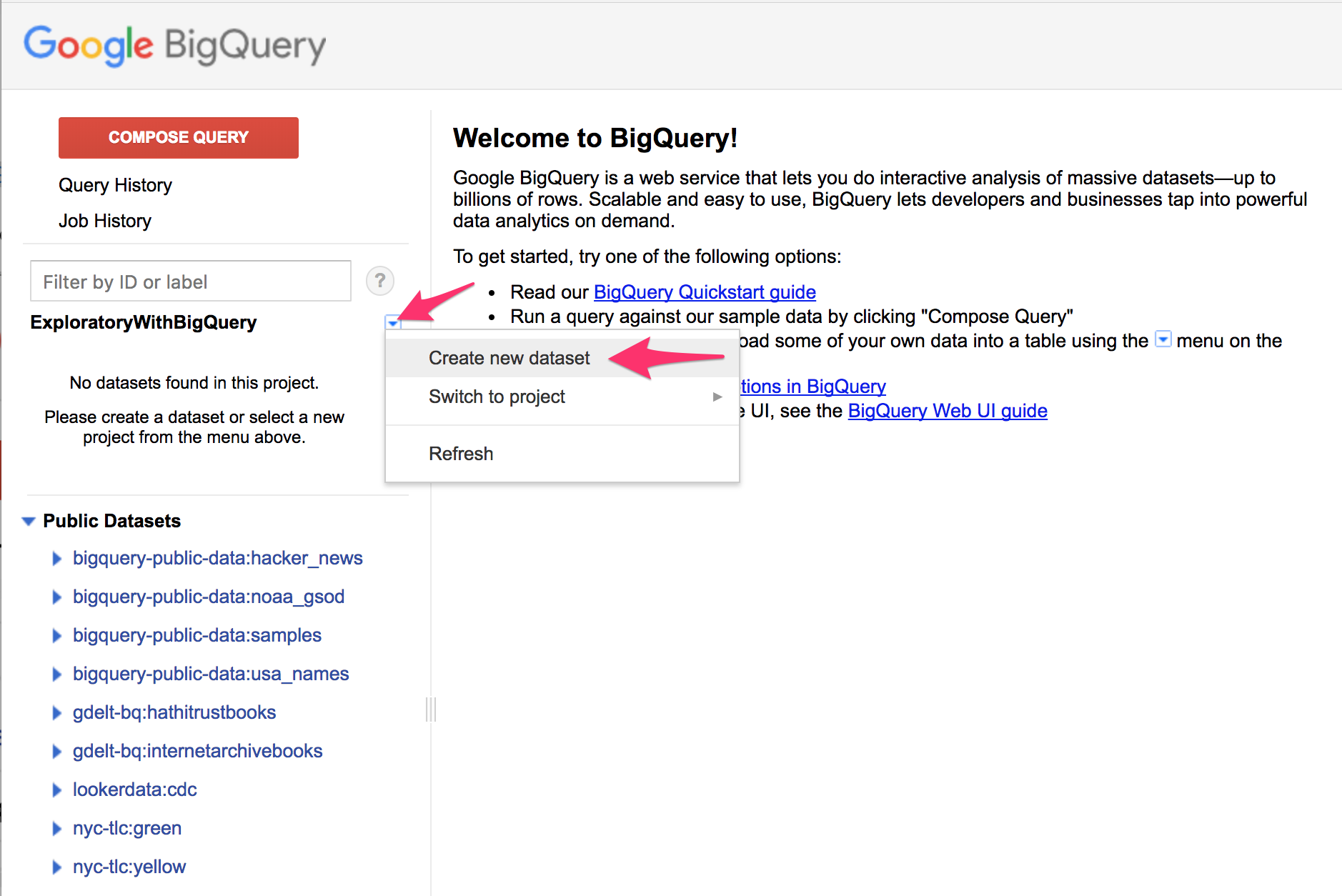The top of the image features a gray banner. On the left, there is a multi-colored Google logo, next to which is black text reading "BigQuery." To the right of this logo, a red button with white text reads "Compose Query." Below this, headlines in black text read "Query History" and "Job History."

A box labeled "Filter by ID or Label" appears beneath these headlines. Following this, the text "Exploratory with BigQuery" is visible. Below this, a message states, "No data sets found in this project. Please create a data set or select a new project from the menu above." Beneath this message, the image lists public data sets in blue text, including:
- BigQuery-public-data-hacker_news
- BigQuery public data samples
- NOAA BigQuery public data
- BigQuery public data USA names
- GDELT-BQ
- HathiTrustbooks

On the right side, text reads, "Welcome to BigQuery." It introduces Google BigQuery as a web service enabling interactive analysis of massive data sets, up to billions of rows. The service is described as scalable and easy to use, meant for both developers and businesses to leverage powerful data analytics on demand. The text suggests getting started by reading the "BigQuery Quick Start Guide," which is linked, or by running a query against a sample by clicking "Compose."

The rest of the text is obscured by a pop-up box that says "Create New Data Set," which has a red arrow pointing to it and a drop-down button also indicated by a red arrow. The pop-up includes options such as "Switch to Project" and "Refresh."